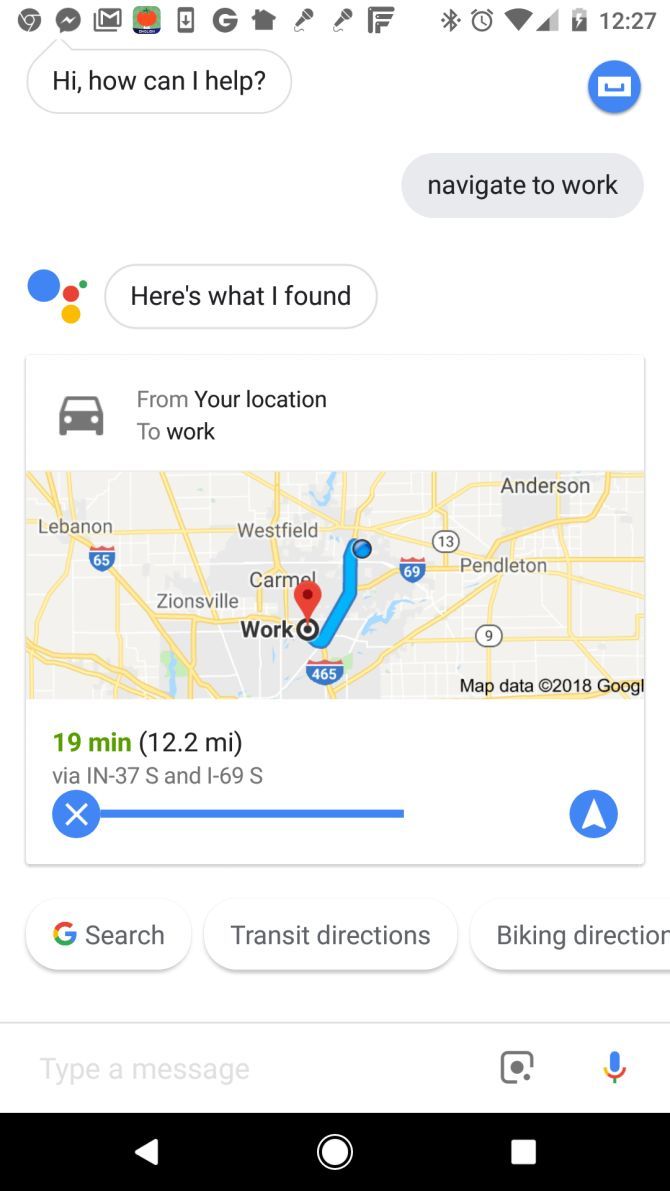This screenshot captures a detailed view of a text message conversation between a user and Google AI on a smartphone. At the top of the screen, standard phone interface elements are visible, including notification icons, the current time, battery level, and network status. At the bottom of the screen, the typical navigation bar includes icons for the homepage, the 'back' button, and a 'close all apps' option.

The conversation starts with Google AI greeting the user with, "Hi, how can I help?" The user then requests, "Navigate to work." In response, Google AI provides a detailed map showing the route from the user's current location to their workplace. The map highlights the pathway, estimating the travel time to be 19 minutes for a distance of 12.2 miles. The route primarily follows Interstate 37 South and Interstate 69 South.

Additionally, the interface includes tags for quick access to 'Google Search,' 'Transit Directions,' and 'Biking Directions.' Below the conversation, there is an input field for the user to continue interacting with the AI. The overall design is intuitive, ensuring seamless navigation and clear communication between the user and the AI.